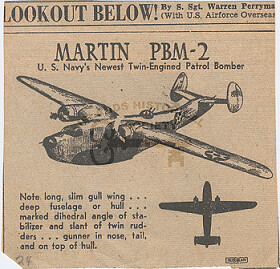This detailed and weathered page, likely a cutout from an old instruction manual or military pamphlet, features a striking illustration and specifications of the Martin PBM-2, the U.S. Navy's newest twin-engined patrol bomber at the time. The page, aged to an orange-brown hue, showcases a large, carefully drawn image of the aircraft. Above the image, the title "Look Out Below" by S. Sergeant Warren Perriman, U.S. Air Force Overseas, commands attention. Below the main image, a smaller overhead view provides additional perspective. The text around the illustration emphasizes notable features of the aircraft: "Note long, slim gull-wing, deep fuselage or hull, marked dihedral angle of stabilizer and slant of twin rudders, gunner in nose, tail, and on top of hull." A shadowy depiction of the plane adds further detail. The bottom left corner is marked with the number 24 in pencil, adding to the artifact's historical intrigue.